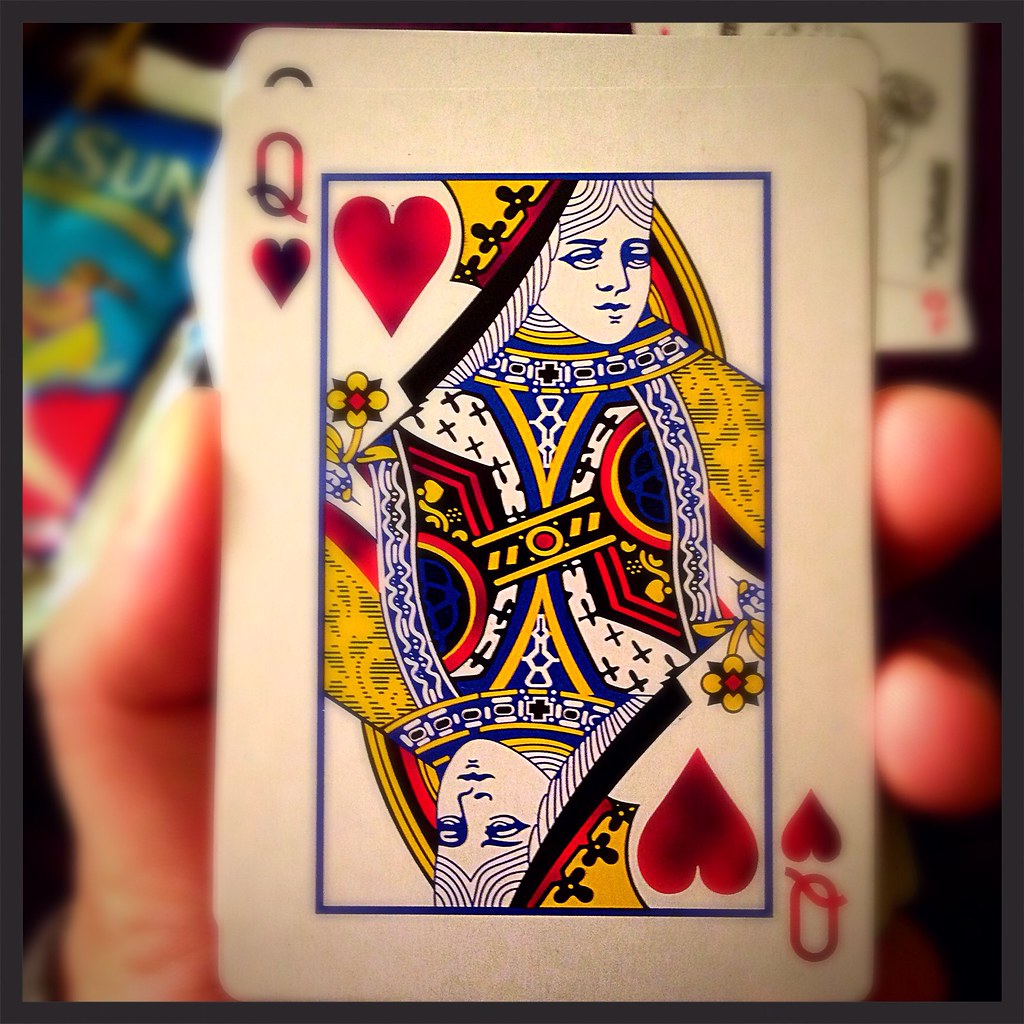This photograph features a close-up of a playing card, specifically the Queen of Hearts, held by a hand emerging from the lower left corner. The card shows intricate detailing: a red-printed Queen adorned in a yellow cape with blue decorations over a white shirt, and a blue border accentuating the central image. The Queen's face is oriented to the right at the top and to the left at the bottom. The image is framed in a square format with a dark grey border. The background is notably blurred, adding a sense of depth to the composition. In the left part of the background, there is a small Sunny Delight juice packet with a blue label featuring the word "Sun" across the top and a yellow stripe. The packet is predominantly red at the bottom and angled to the right, with a visible straw emerging from the top. On the right side, near the upper edge, an indistinct white square object can be seen in the blurred backdrop.